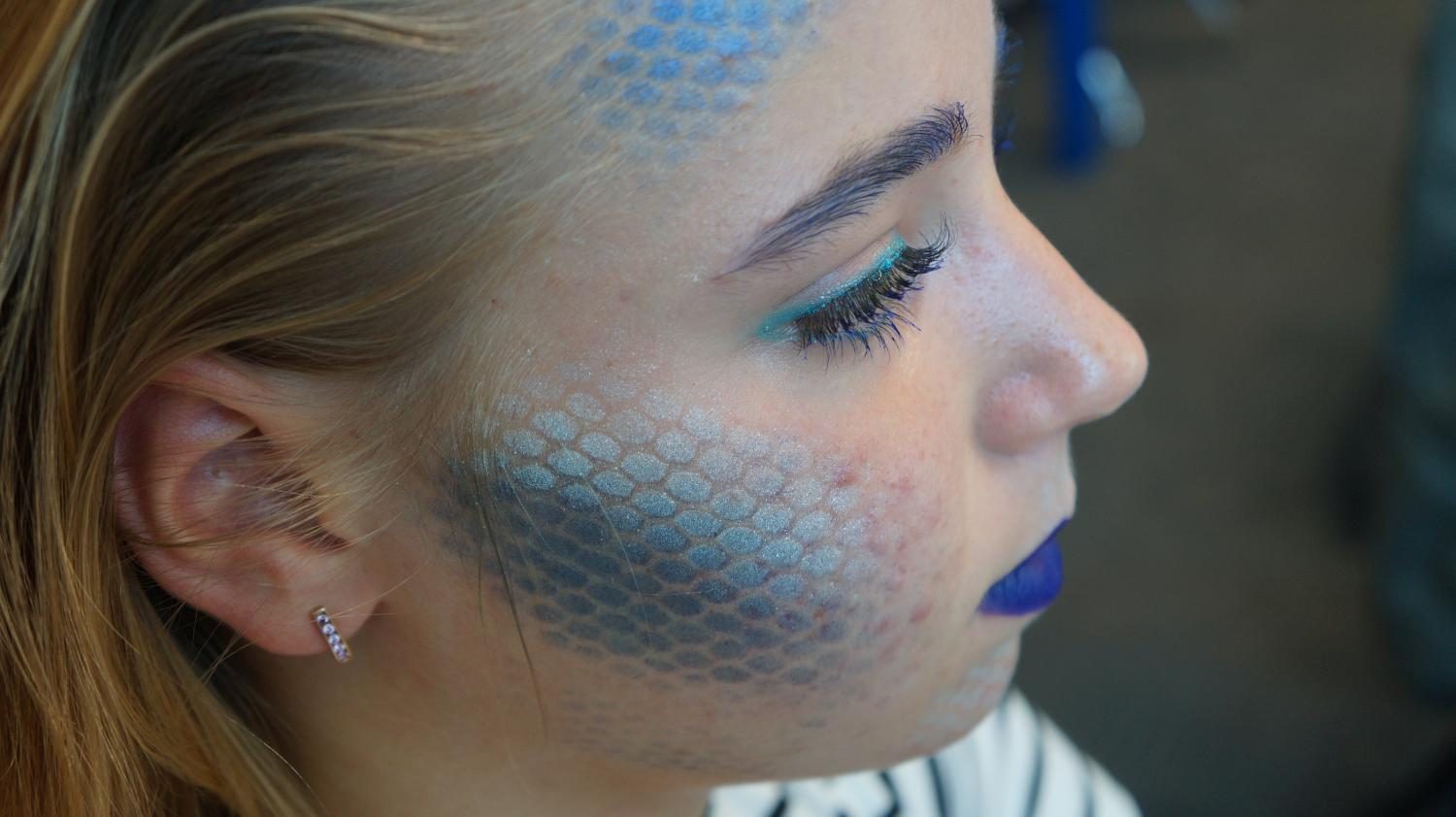The photograph is a detailed close-up of the right side of a young girl’s face, who appears to be around 12 years old. The background of the image is blurry, drawing focus to her facial features. The girl has long blonde hair and is seen wearing a white and black striped shirt. Her face is elaborately decorated with face paint designed to resemble scales, giving her a fantastical, mermaid-like appearance. The scales, crafted from shimmering blue dots, cover her cheeks and forehead, blending into her skin with a silvery, sci-fi effect. 

Her eye makeup includes blue eyeshadow with light blue on the top and dark blue on the bottom, along with blue-enhanced eyebrows and extended eyelashes. She sports blue lipstick that complements the shimmering scales. Her ear is visible, adorned with a small hoop earring featuring clear gemstones. The overall effect is a transformative, enchanting look reminiscent of a mystical sea creature.